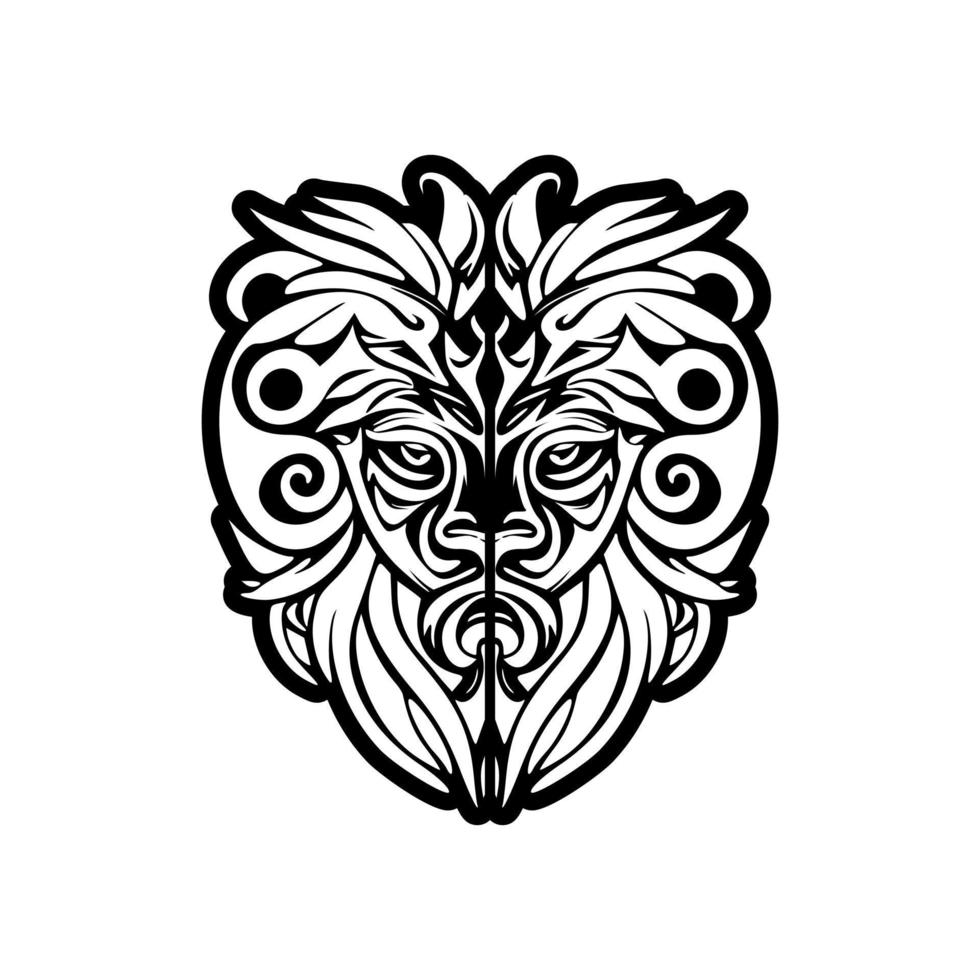The image is a black-and-white drawing against a white background, featuring an intricate and stylized lion-like creature. Its face, prominently outlined in bold black lines, sports dark, triangular pupils and thick eyebrows. The creature's nose is wide and solid black in color. Surrounding the face, the hair is depicted with sharp, spiky tendrils in the center that curve and protrude upward, while the sides feature curly strands. The creature's distinctive facial hair includes a long, drooping mustache and a thick, tendril-lined beard. The absence of any background enhances the boldness of the creature's visage, suggesting its suitability for a tattoo stencil design, with its purely black and white palette accentuating the striking contrasts.